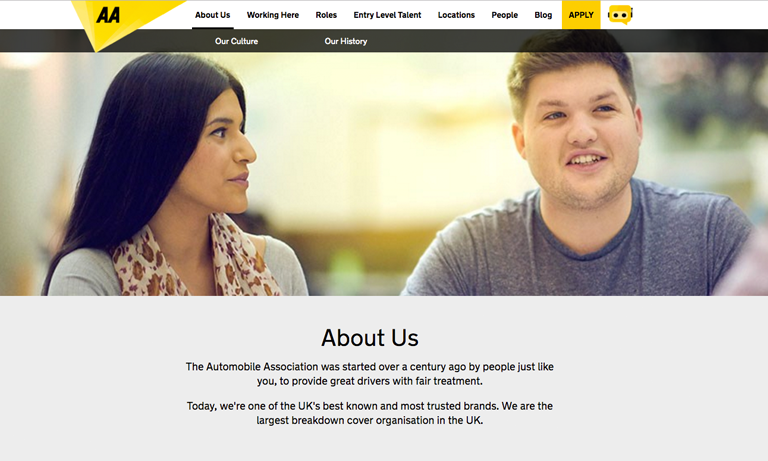The image depicts a webpage prominently featuring a horizontally aligned banner occupying the upper half. This banner showcases a side profile of a woman on the left, who has long black hair and is adorned with a patterned white and brown scarf around her neck. To the right stands a man clad in a grey t-shirt. Below this engaging visual, text reads: "About Us: The Automobile Association was started over a century ago by people just like you to provide great drivers with fair treatment. Today, we are one of the UK's best known and most trusted brands. We are the largest breakdown cover organization in the UK."